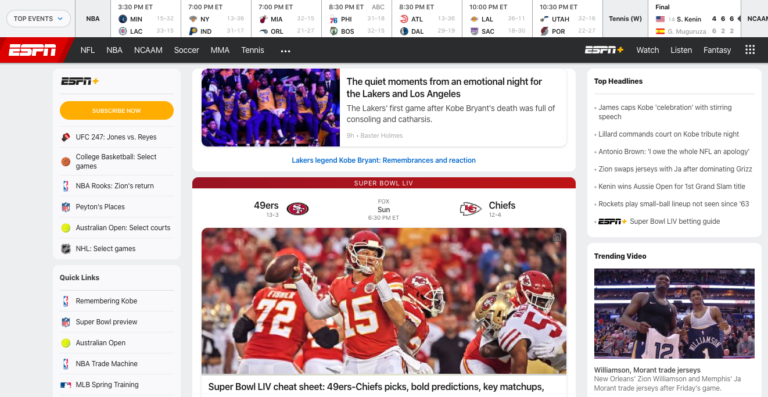In this detailed screenshot from the ESPN website, the image captures various elements starting at the top of the page. At the very top, we see scoreboards detailing several NBA games along with their start times, spreading across the top banner. In the top right corner, the page transitions to display the final score of a completed tennis match.

Adjacent to the tennis scoreboard, an NCAA section appears, though it is unclear if the content pertains to basketball or football. Beneath these scoreboards, the iconic ESPN logo is prominently displayed on the left side in its familiar red and white colors.

Parallel to the logo on the right side of the black navigation bar, several menu tabs are visible, including NFL, NBA, NCAA (Men's Basketball), Soccer, MMA, Tennis, ESPN+, Watch, Listen, and Fantasy.

Below this navigation bar, a column of articles is presented against a white background on the left side. Dominating the center of the page is an eye-catching feature about the Super Bowl, highlighting the thrilling matchup between the San Francisco 49ers and the Kansas City Chiefs. The featured image shows Patrick Mahomes, quarterback for the Chiefs, captured in action as he throws a football during the game against the 49ers.